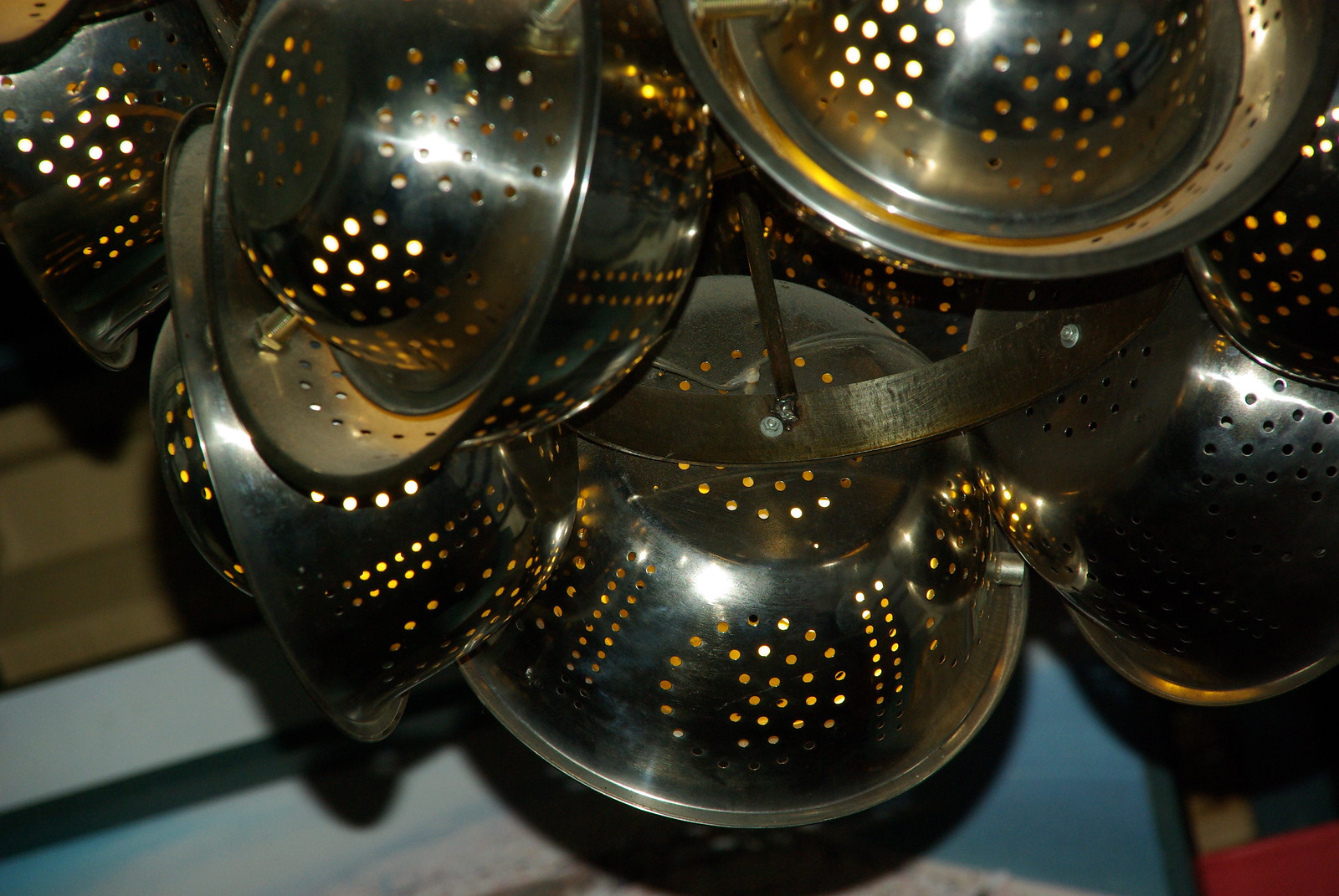The image showcases a striking modern art chandelier made from multiple hanging metal colanders of varying sizes. These colanders, repurposed into an artistic display, feature intricate patterns of holes in the shapes of I's and O's along their sides and bottoms. They are affixed with screws and rods to a large circular metal rack, effectively grouped together. An orange light shines through the colanders, casting a golden reflection where the light hits and creating a warm glow. The chandelier is suspended over a wooden floor near a light brown countertop, accompanied by a light blue low wall and dark-colored cabinets in the background. A red chair is also noticeable in the scene, but the centerpiece is undoubtedly the ingeniously crafted chandelier that transforms everyday kitchen implements into a piece of contemporary art.